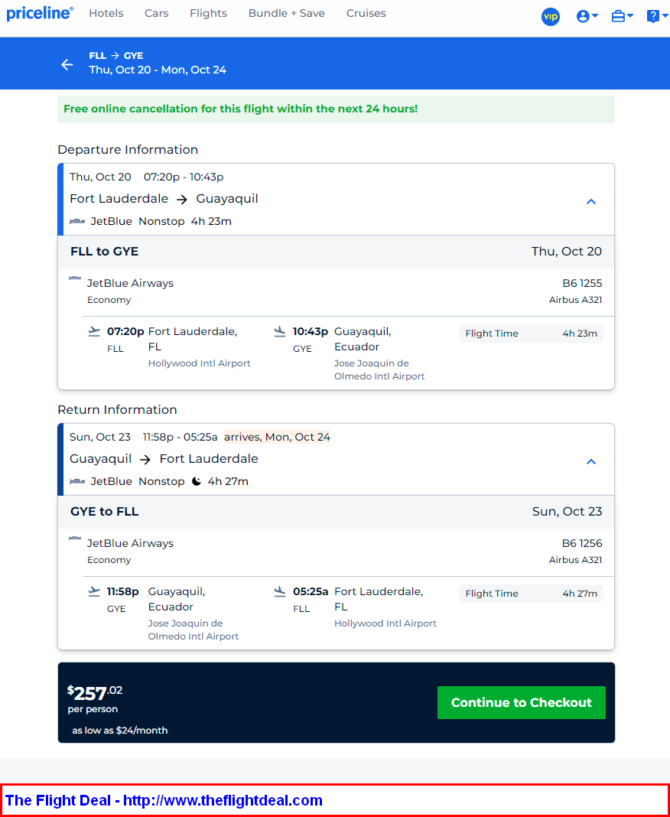Screenshot of a Travel Booking Website

The screenshot captures a travel booking website with a predominantly white background accented by blue, green, and black. 

**Header Section:**
- **Top Left Corner:** The site name "priceline" is displayed in lowercase blue font.
- **Top Center:** Navigation options in black, smaller font include "hotels," "cars," "flights," "bundles and save," and "cruises."
- **Top Right Corner:** User initials, a profile drop-down box, and two icons resembling a cake and a question mark are visible.

**Main Content:**
- **Blue Bar:** Spanning the width of the site, it displays flight details: "Thursday October 20th to Monday October 24th."
- **Green Alert Box:** Slightly pale green background with the message "Free online cancellation for this flight within the next 24 hours."

**Flight Information:**
- **Departure Details:** Provides the departure date, airport of departure and landing, airline name, and flight duration (non-stop, 4 hours and 23 minutes).
- **Return Information:** Mirrors the departure details in reverse.

**Footer Section:**
- **Price and Action Button:** A black box at the bottom displays the total price of $257 per person in white font. Adjacent to it is a green button labeled "continue to check out."
- **Additional Note:** At the very bottom, a red-outlined box contains a blue text link to a flight deal website: "The Flight Deal - http://www.theflightdeal.com."